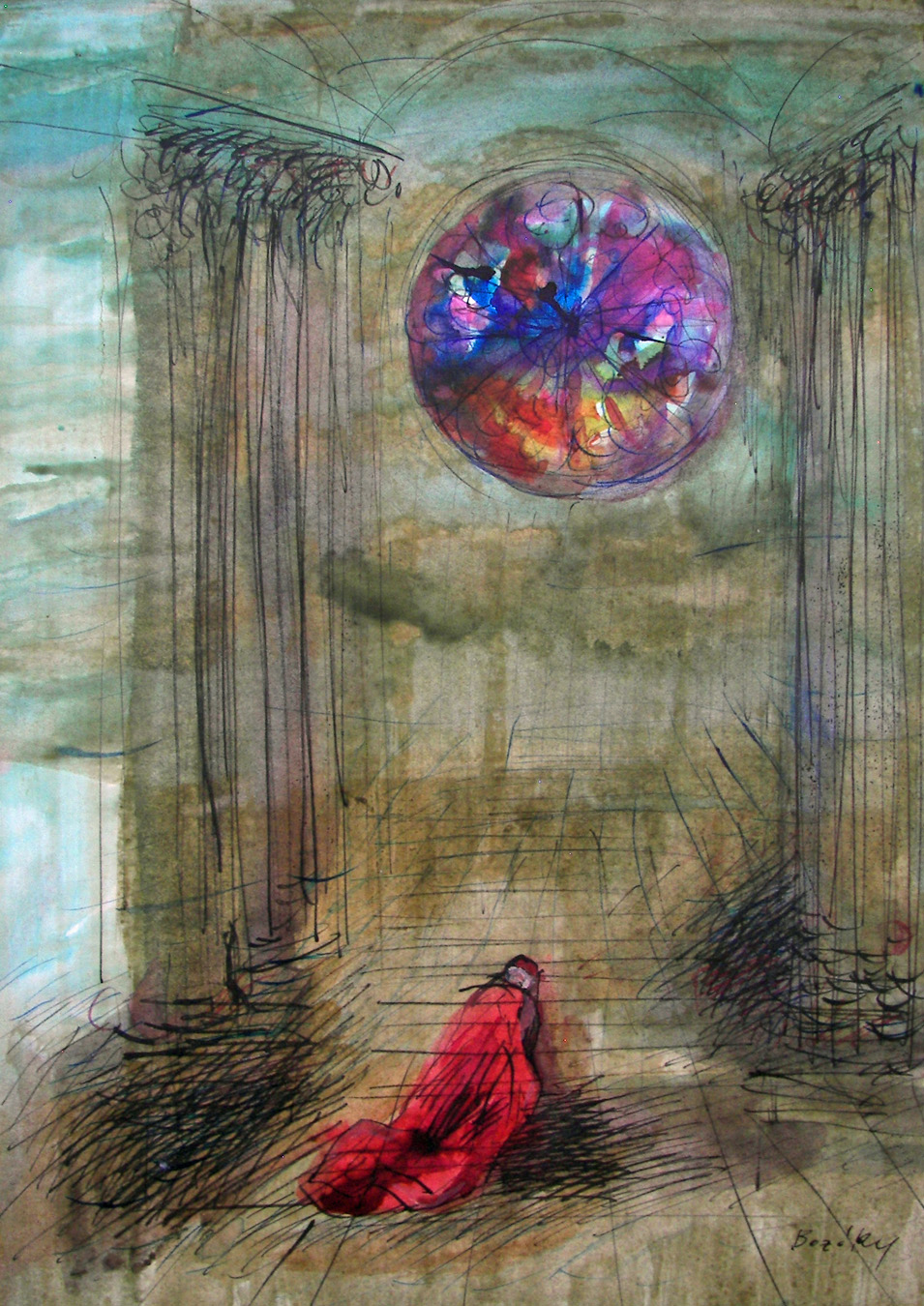The image depicts a watercolor painting with ink drawing detailing. It illustrates a man in a bright red cape or robe, kneeling or crawling on the ground, surrounded by what appears to be broken sticks. The individual is moving away from the foreground. The background features a large, round stained glass window, centered at the top of the image. This window is vividly colored, showcasing a vibrant spectrum of blues, purples, pinks on the top half, and oranges, yellows, and reds on the bottom half. The whole design is encased in a rounded arch. On either side of the window are towering columns that stretch from the bottom to the top of the painting. The overall environment hints at a cathedral-like setting, though it's unclear if it's indoors or outdoors due to the sketchy nature of the artwork. The cathedral's structure is depicted with drab browns and greens, contrasting with the vivid stained glass. The artist's signature is located at the bottom right, beginning with a 'B' and ending with a 'Y', though the exact name is difficult to discern, possibly Beasley or Beadley.